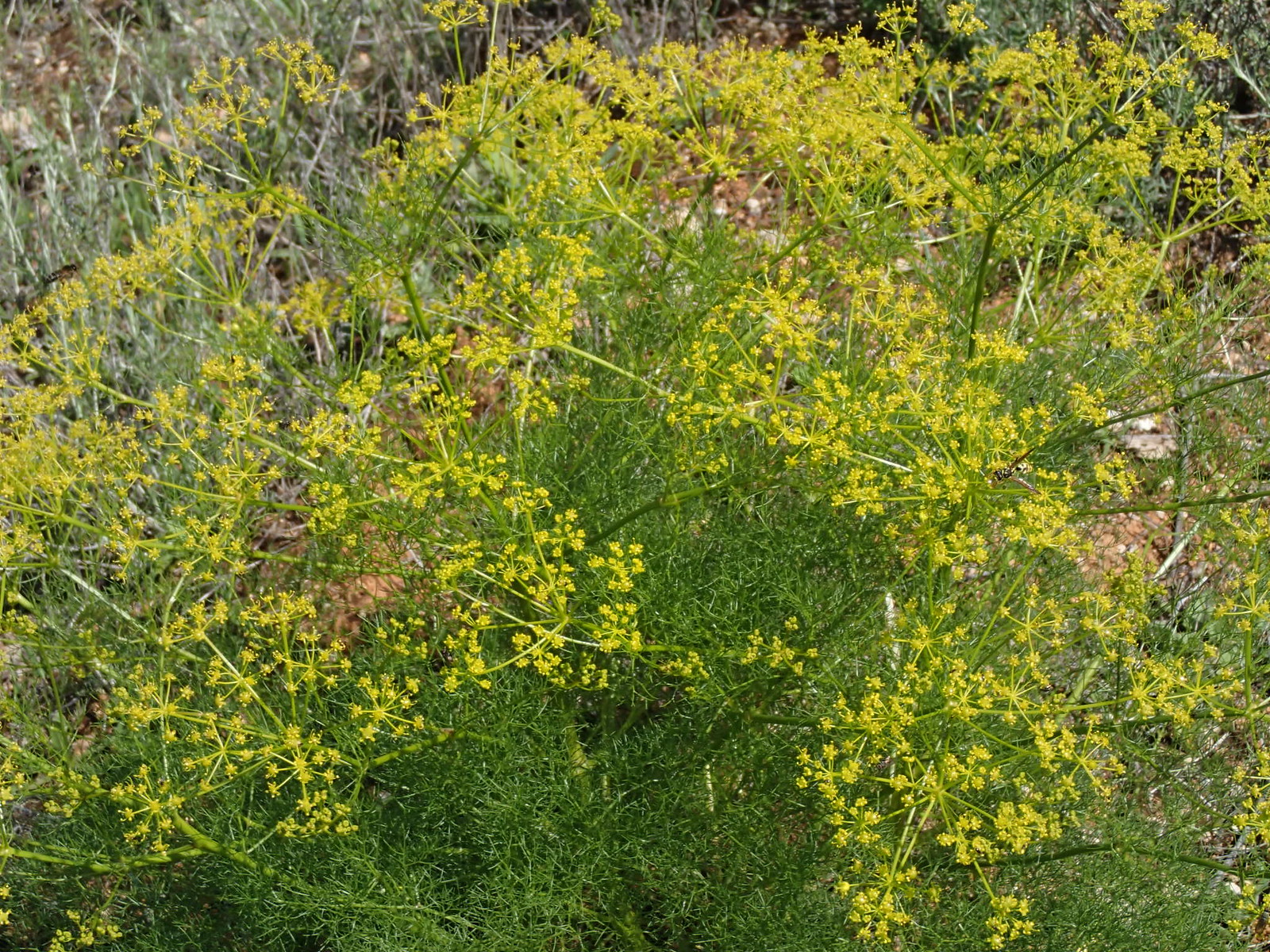The photograph showcases a large, vibrant green plant densely populated with tiny, bright yellow wildflowers clustered at the ends of thin stems. The plant dominates the image, creating a striking contrast between the lush greenery and the vivid yellow flowers. The backdrop reveals a rocky, possibly tan terrain that is somewhat blurred and indistinct, lending a rugged context to the scene. Additional elements in the background include more arid, grayish, or light brown dead branches that lack leaves, especially noticeable in the top left corner. These dried weeds and branches further highlight the healthy, flourishing state of the main plant in the foreground, which stands out as the focal point against the otherwise sparse and rocky environment. The sky is not visible in the photograph, keeping the focus entirely on the interplay between the living and dead vegetation within this outdoor setting.